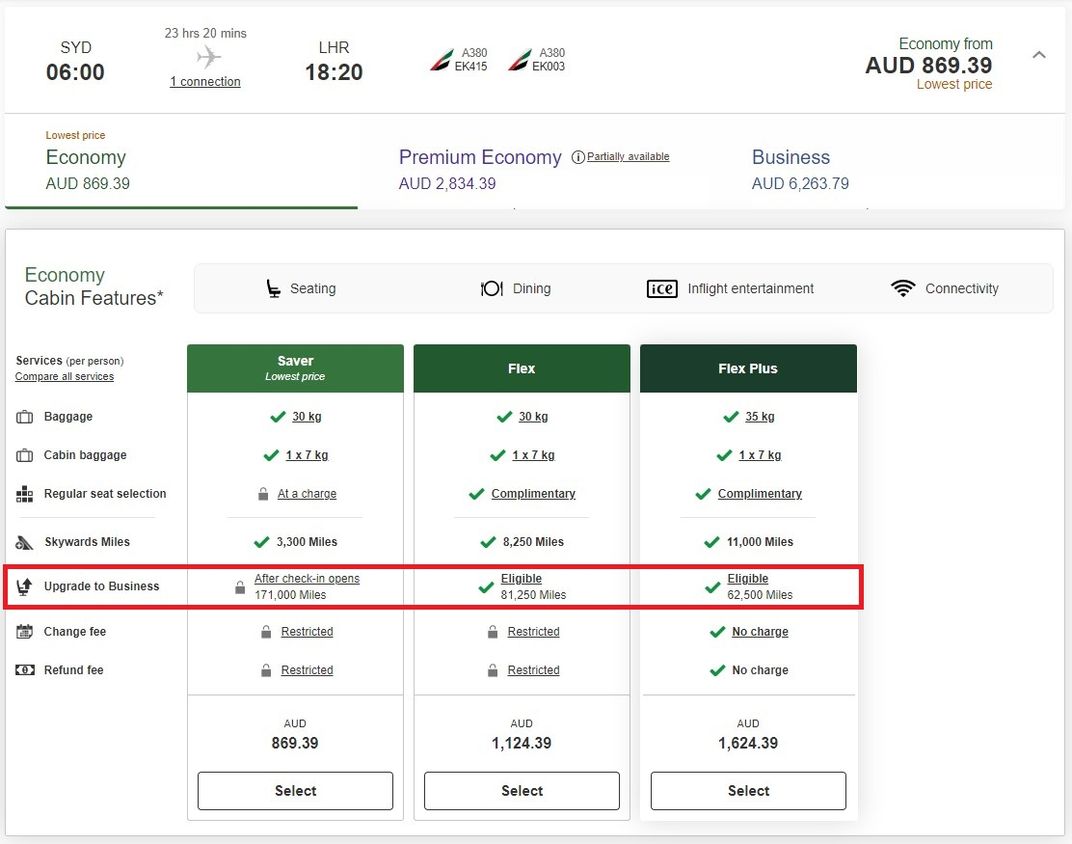Screenshot Caption:

The screenshot depicts a detailed itinerary and pricing breakdown for a flight from Sydney to London Heathrow (LHR). The flight includes information about different travel classes and their respective prices in Australian Dollars (AUD). 

In the upper right corner, the lowest price displayed is AUD 869.39 for economy class. The itinerary details include a departure from Sydney at 6:00 and arrival in London at 18:20. The journey involves one connection, and the aircraft used for the flight segments are both Airbus A380s.

The pricing for different travel classes is as follows:
- Economy: AUD 869.39
- Premium Economy: AUD 2,834.39
- Business: AUD 6,263.79

For the Economy cabin, there are three fare options:
1. Saver:
   - Baggage allowance: 30 kg
   - Cabin baggage: 1 x 7 kg
   - Regular seat selection (for an additional charge)
   - Dining
   - In-flight entertainment
   - Connectivity
   - Skywards miles earned: 3,300 miles

2. Flex:
   - Baggage allowance: 30 kg
   - Cabin baggage: 1 x 7 kg
   - Complimentary dining
   - Connections similar to Saver
   - Skywards miles earned: 8,250 miles

3. Flex Plus:
   - Baggage allowance: 35 kg
   - Cabin baggage: 1 x 7 kg
   - Complimentary seat selection
   - Dining
   - In-flight entertainment
   - Connectivity
   - Skywards miles earned: 11,000 miles
   - Note: Eligible for an upgrade to business class after check-in, subject to charge and change fee.

At the bottom of the screenshot, the total fares for each option are summarized:
- Saver: AUD 869.39 (matching the estimate in the upper right corner)
- Flex: AUD 1,124.39
- Flex Plus: AUD 1,624.39

The screenshot comprehensively covers various pricing, seating, and service options for a flight from Sydney to London Heathrow.